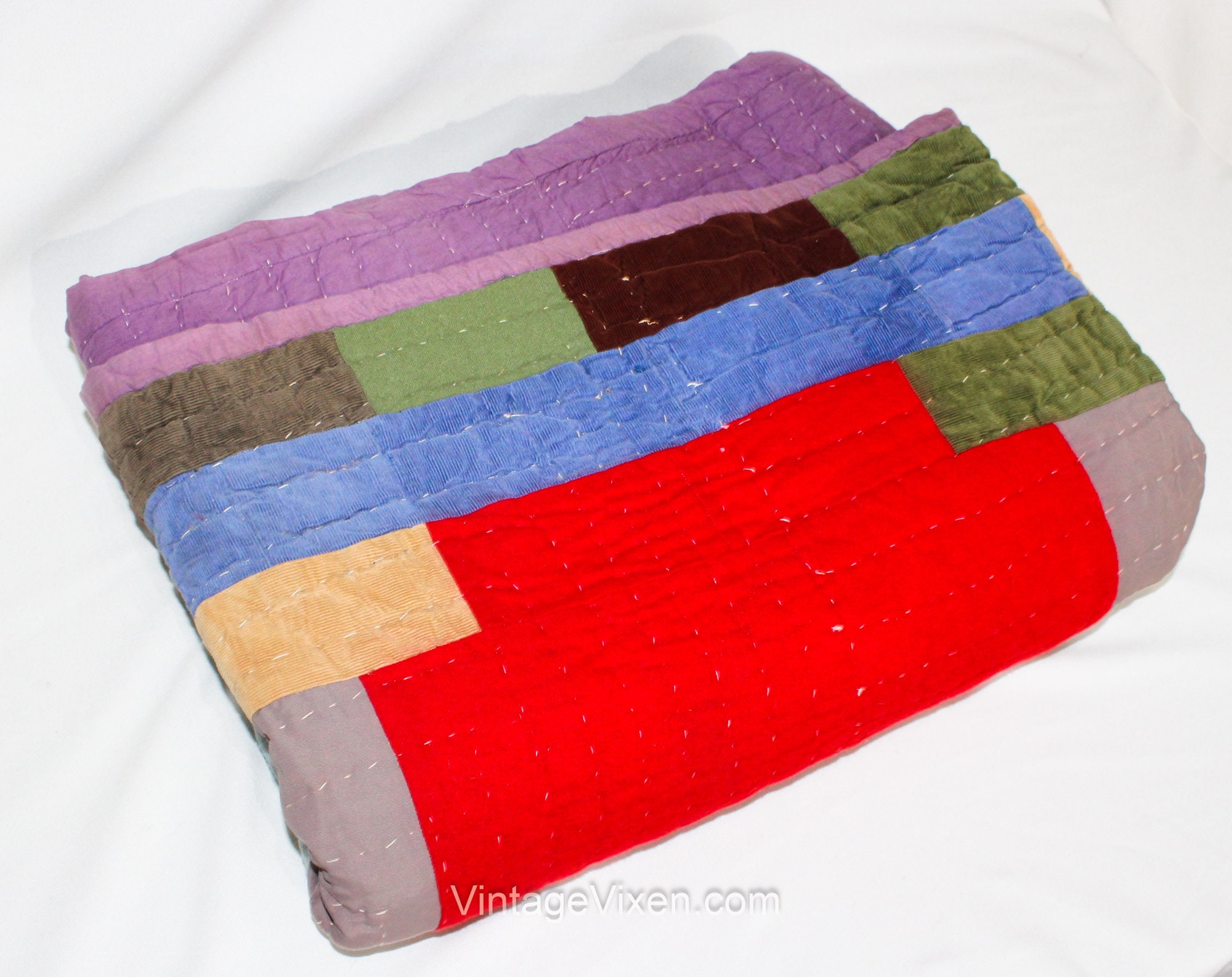The image features a vintage, folded quilt resting on a white fabric surface, possibly a bed. The quilt showcases a color-block design with a variety of rectangle shapes in an array of colors, including dark green, light green, black, army green, blue, red, gray, dark and light purple, and a yellowish-orange hue. Each colored section is stitched with white thread, enhancing its detailed look. The visible edges of the quilt prominently display dark and lavender purples. Below those, there are rows of alternating rectangles: dark green, a normal green, a dark brown line, and a dark forest green. Further down, there's a sequence with blue-colored rectangles, some being slightly darker, followed by a row featuring red in the center, yellow on the left, and forest green on the right. The bottom edge of the quilt transitions from red to gray, reinforcing its antique charm. The entire piece, folded into a square, emphasizes its meticulous craftsmanship, and the bottom right corner of the image has the watermark "VintageVixen.com" delicately inscribed.